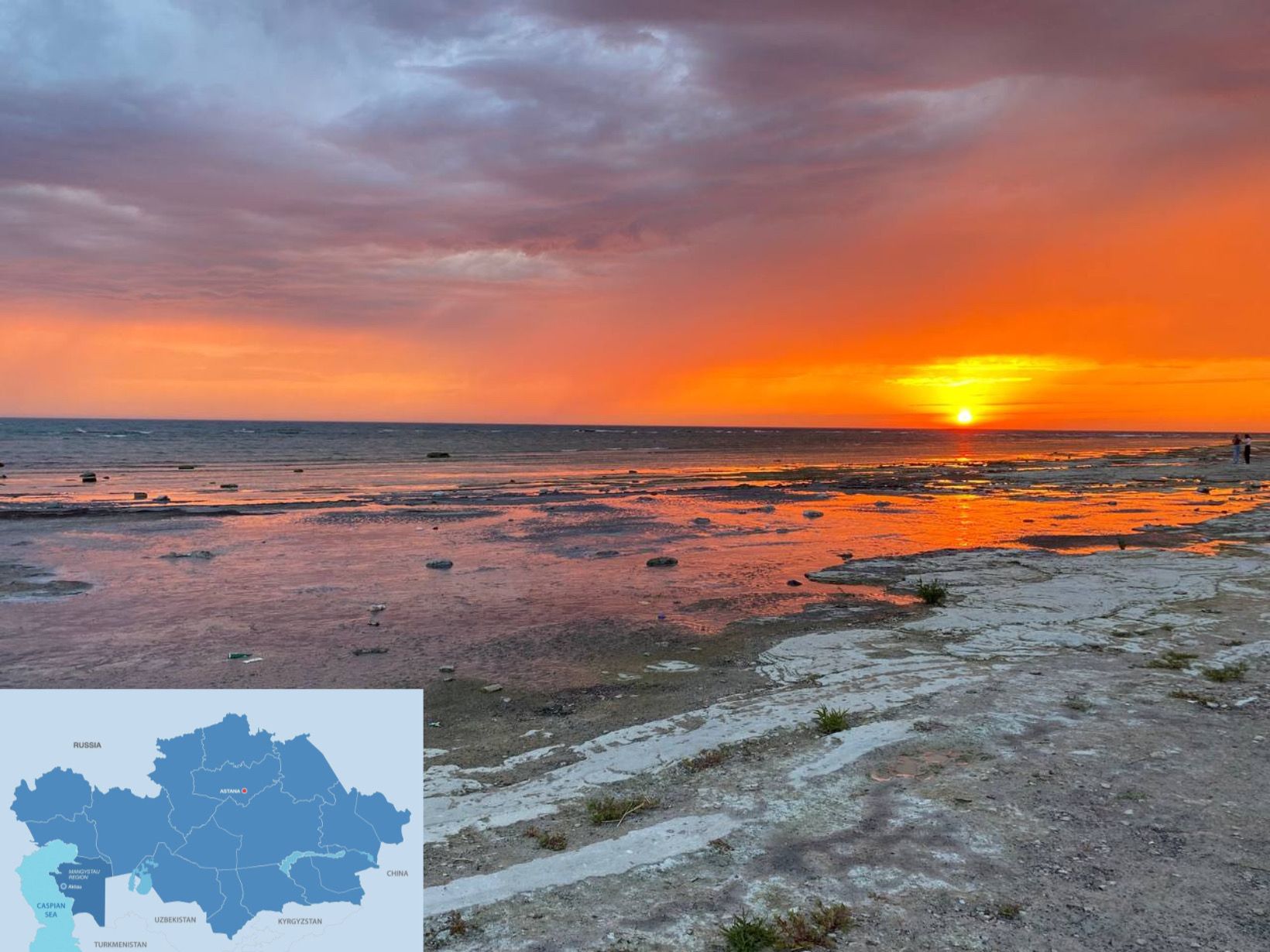In the foreground of this beach scene, a map located in the lower left corner displays indistinct regions against a muted light blue background, possibly indicating various shaded areas, albeit faintly legible due to its small size. Dominating the horizon, the sun is either rising or setting, casting a brilliant orange and yellow glow across the sky, which transitions to gray clouds as they move forward. The beach, composed of gray and white sand, is scattered with patches of grass and a few plants. In the far background on the right side, two people can be seen amidst the rocks along the shore, enhancing the serene ambiance of this coastal landscape.